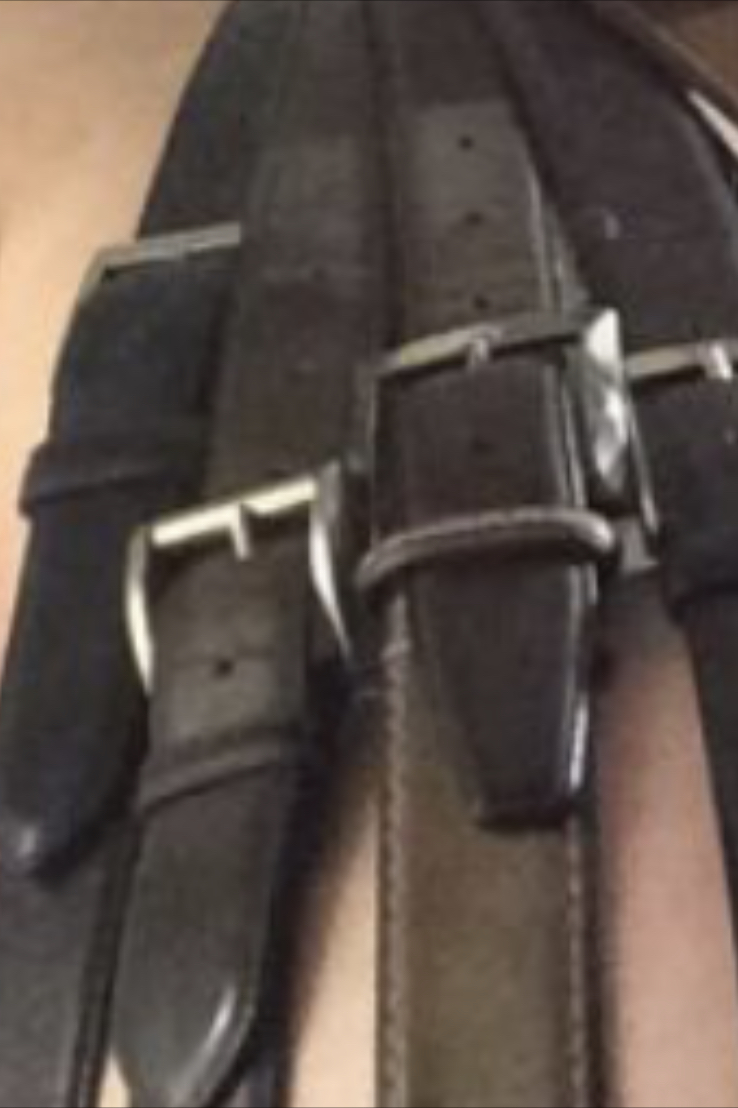This out-of-focus portrait-format photo shows a small collection of worn men's leather belts, hanging vertically and fanning out toward the bottom of the frame. The belts, primarily black with one dark brown, are secured with silver buckle-style hardware and are mostly fastened on the second hole. They appear dusty with signs of use, indicating frequent wear. The ends of the belts are clustered together at the top of the image, while the outermost belts run off the edges of the photo. The belts are set against a nondescript peach flesh-colored background that adds a stark contrast to their darker hues. Despite the image's blurred and low-resolution quality, the worn texture and uniform thickness of the belts are discernible, hinting at a common style and purpose.